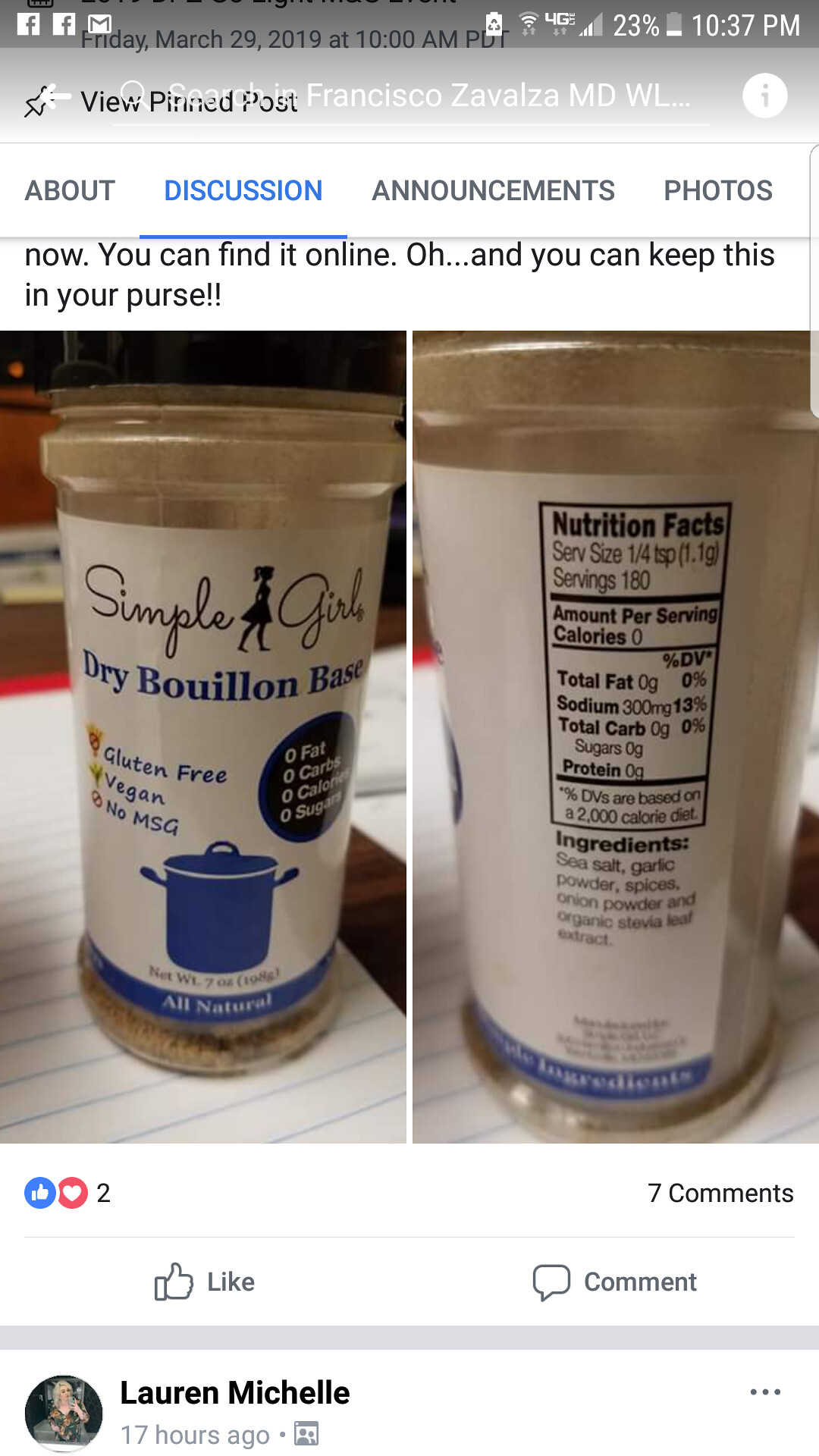The image is a screenshot of a Facebook post taken from a cell phone, evident from the notifications and various icons at the top. The post features two side-by-side photos of a plastic spice container with a black cap and a white, blue, and black label. The left image shows the front of the container, labeled "Simple Girl Dry Bouillon Base," which is gluten-free, vegan, and devoid of MSG, fat, carbs, calories, or sugars. The label includes a silhouette of a woman between the words "Simple" and "Girl." The right image displays the nutritional facts: a serving size of a quarter teaspoon and values indicating zero calories, fat, carbs, sugars, and protein, with 300 mg of sodium. Ingredients listed are sea salt, garlic powder, spices, onion powder, and organic stevia leaf extract. Below the photos, it notes there are seven comments on the post, one from a user named Lauren Michelle, made 17 hours ago. Additionally, the top portion refers to a pinned post about discussion, announcements, and photos, highlighted in blue. There's also a like button and a comment section beneath the post.